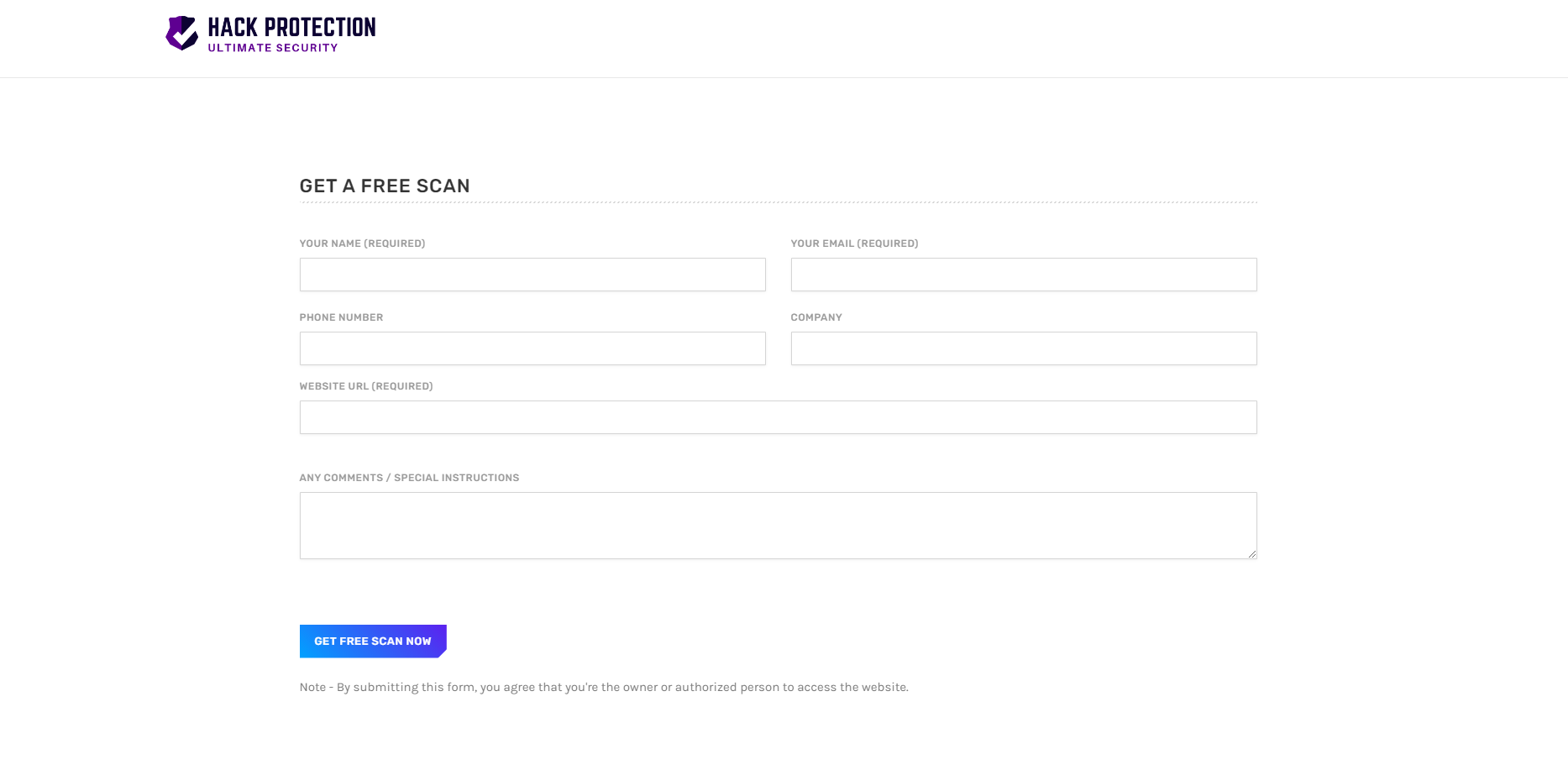The image is a screenshot of an online form designed for a hack protection service. On a white background, the top left corner features a purple shield-shaped icon with a large white checkmark in its center, symbolizing security. Directly to the right, in large black lettering, the text reads "Hack Protection," with the phrase "Ultimate Security" in purple below it.

Under the header, a thin gray line runs across the page, separating it from the main content below. The form begins with a prominent heading in large black text saying, "Get a Free Scan." This is followed by several text fields intended for the user to fill out:

- "Your Name" (required) – currently blank
- "Phone Number" – currently blank
- "Website URL" (required) – currently blank
- "Any Comments/Special Instructions" – a comment section at the bottom, also blank

On the right side of the form, additional fields are displayed:

- "Your Email" (required) – currently blank
- "Company" – currently blank

At the very bottom left corner, there is a rectangular button that transitions from blue on the left to purple on the right. In bold, white, uppercase letters, it reads "Get Free Scan Now." Below this button, a note in black text states, "By submitting this form, you agree that you are the owner or authorized person to access the website."

This form appears minimalistic yet functional, aimed at obtaining essential information from users seeking a security scan for their websites.